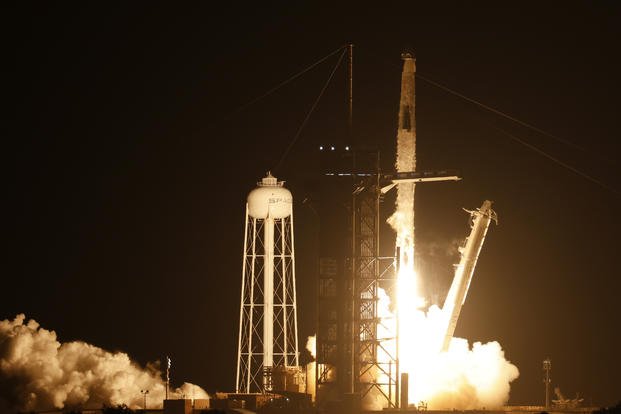This image captures the dramatic nighttime launch of a small, thin rocket. The rocket, which is ascending into the dark sky from the center of the photo, leaves a trail of fire and smoke at its exhaust. A metal scaffolding structure with numerous cables, from which the rocket has just detached, dominates the central vertical axis of the image. To the right of the scaffolding, you can see the fallaway platform descending after the liftoff. On the left side of the image, a tall white water tower stands prominently, with another similar tower visible in the distant background. A thick cloud of white smoke collects at the bottom left corner, partially obscuring a flag positioned in front of the plume. Numerous buildings are visible at ground level, silhouetted by the bright explosion at the rocket's base. The entire scene is enveloped in darkness, highlighting the luminous elements of the rocket's ascent.